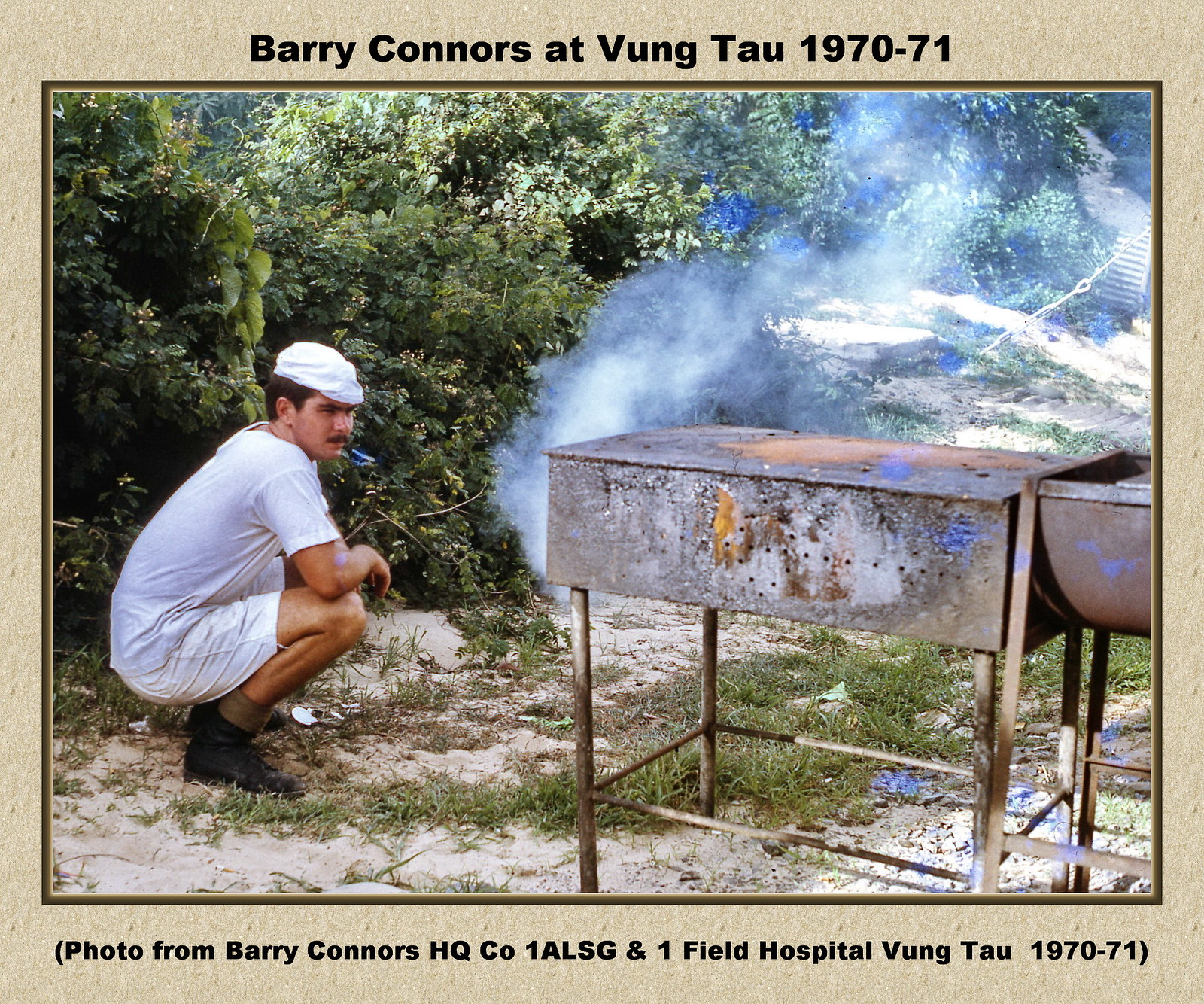In this vintage photograph from the Vietnam War era, dated 1970 to 1971, a white man identified as Barry Connors is captured outdoors, crouching on sandy and grassy terrain. He is dressed in a white hat, a white t-shirt, white shorts, brown socks, and black shoes. Barry appears focused as he looks to his right at an old, beat-up, rusty grill or smoker emanating smoke, suggesting he's cooking something. The background is rich with tree foliage. The image features captions at both the top and bottom: "Barry Connors at Vung Tau" at the top, and, "Photo from Barry Connors HQ Company 1 ALSG and 1 Field Hospital, Vung Tau" at the bottom.